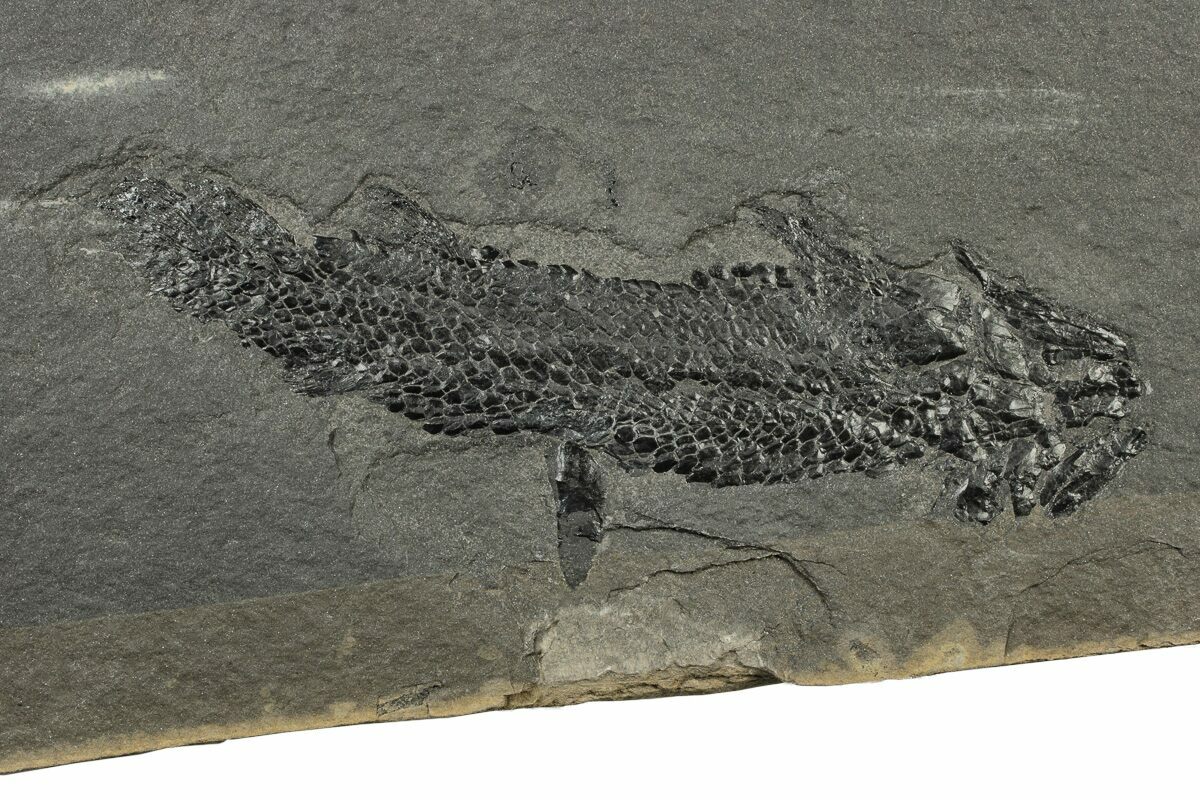The photograph displays a fossil embedded in an old, gray stone, showing a detailed scaly texture and spanning horizontally from left to right. The fossil, slightly darker than the surrounding rock, has a notable sheen and appears to be a fish with an indistinct head and tail. Positioned about halfway along the bottom of the fish, a single fin points downward. The stone features a lighter, browny-beigey area at the bottom, which transitions to an orangish line along the border. The stone itself is cracked near the bottom edge, which angles up to the right, and the overall image includes subtle white streaks scattered across the middle and top areas.